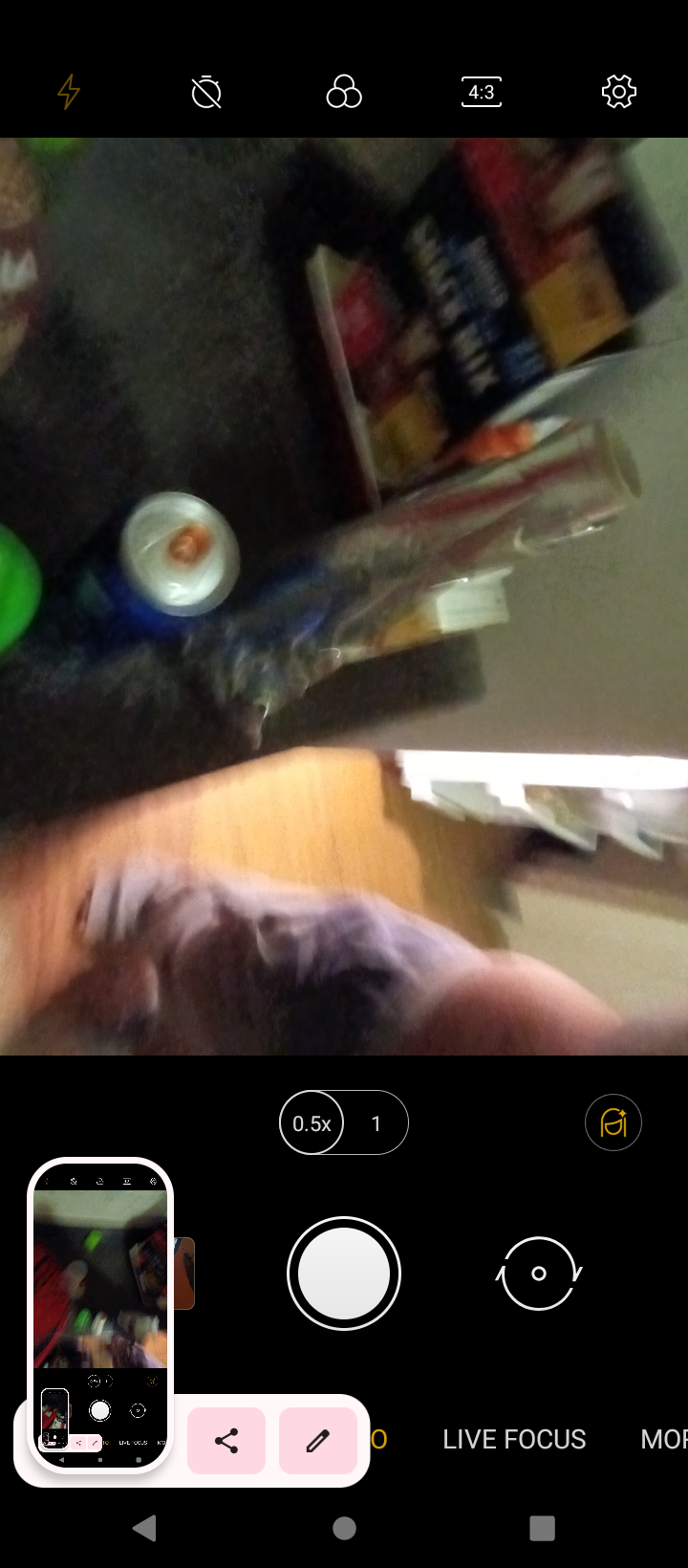The image appears to be a cell phone screenshot capturing a messy cutting board surrounded by various food packages. The cutting board is cluttered with an assortment of items including the top of a metal can and various kinds of food packaging. On the screenshot, the camera's 'Live Focus' mode is indicated at the bottom, along with the camera button. The screen displays black bars at the top and bottom, with several icons visible at the top. The overall scene captures a moment of meal preparation or kitchen activity.